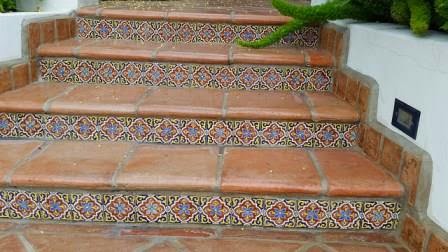The image depicts an aged, decorative staircase seemingly located at a house. The stairs feature faded, orangish-brown clay tiles on their treads, suggesting wear and time. Each riser of the staircase is adorned with a colorful ceramic tile mosaic, showcasing a geometric, diamond-shaped pattern with intricate designs and colors including reds, blues, whites, and blacks. This motif adds a vibrant contrast to the worn steps. The staircase, which consists of about five steps, is framed by white walls on both sides. A lush green plant or vine intrudes from the upper right corner, adding a touch of nature to the scene. Additionally, a small rectangular box, possibly housing an outlet, is visible in the bottom right corner.